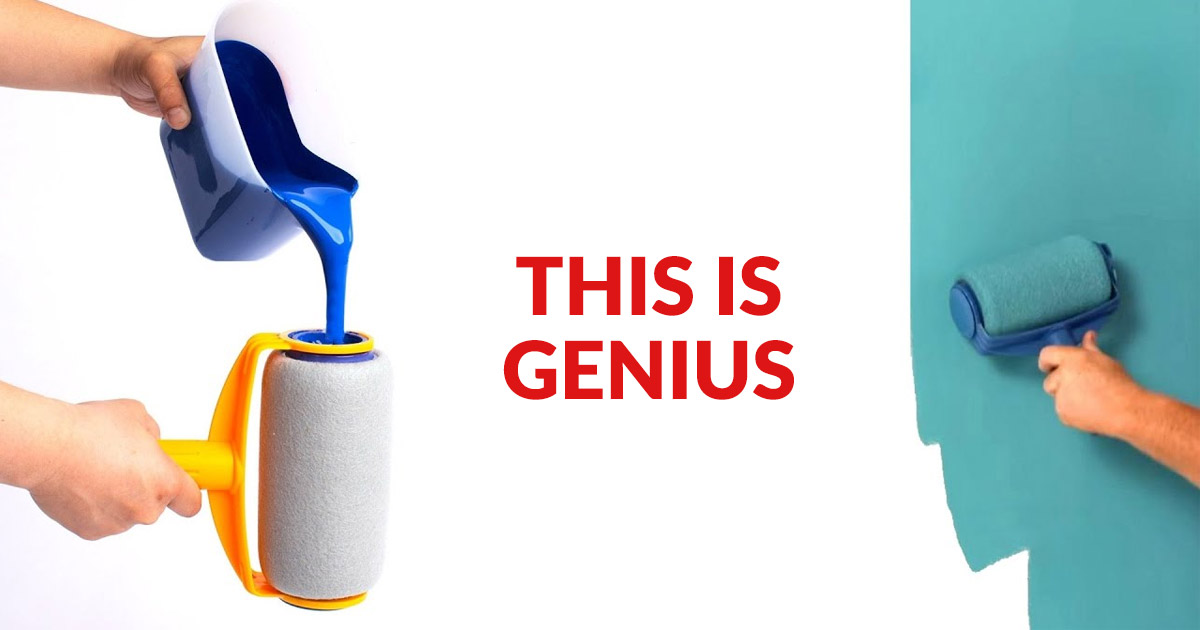The image is a photographic advertisement showcasing an innovative paint roller. It consists of two photographs on a white background with bold red capital letters in the center reading, "THIS IS GENIUS." 

On the left side, a hand holding a yellow-handled paint roller is visible. The roller, which is off-white, has a mechanism designed to be filled with paint directly. Another hand pours bright blue paint from a plastic container into the center of the roller, illustrating the paint-holding capability of the roller.

On the right side, a similar blue-handled roller is being used to spread green paint on a wall. The roller dispenses paint through its fabric, effectively painting the surface. A forearm and hand are shown holding the roller, demonstrating its use. The advertisement emphasizes the roller's efficiency and innovative design for dispensing paint smoothly and continuously.